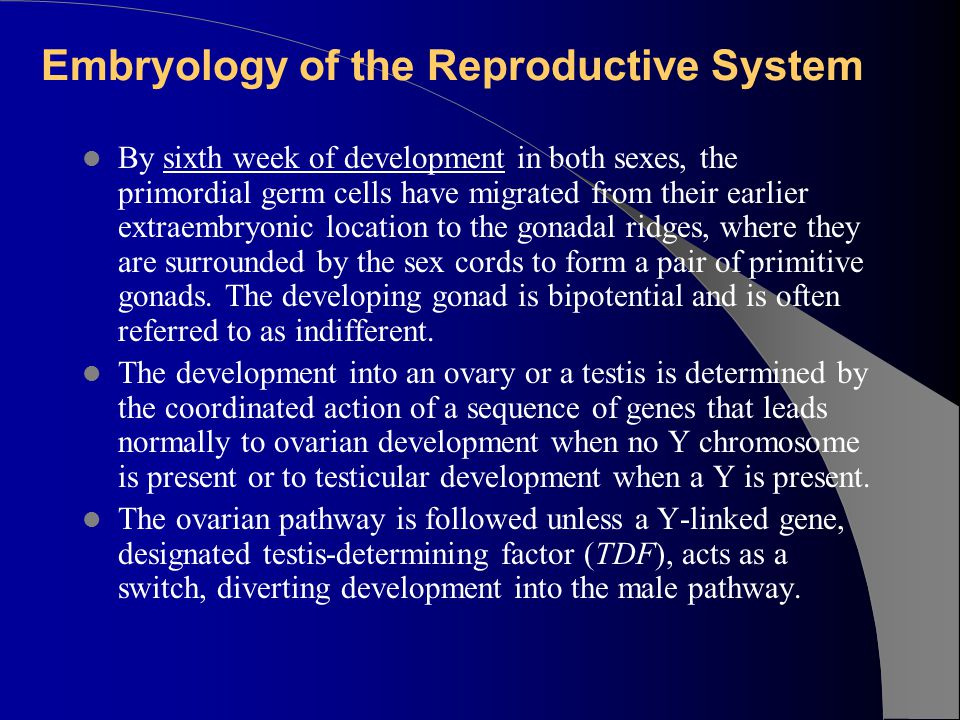The rectangular image, slightly wider than it is tall, features a predominantly text-based design with a background transitioning from royal blue on the left to almost black on the right. This gradient is interrupted by a gray path that starts in the lower right, appearing wide at first, and then curves upward and left, tapering into a thin line near the top left. At the top of the image, in large pale yellow or gold text, it reads "Embryology of the Reproductive System." Below this title, the content is organized into three bullet points filled with detailed text.

The first bullet point, indicated by a gray dot, spans six lines and reads: "By the sixth week of development in both sexes, the primordial germ cells have migrated from their earlier extraembryonic location to the gonadal ridges where they are surrounded by the sex cords to form a pair of primitive gonads. The developing gonad is bipotential and is often referred to as indifferent."

In the second bullet point, also marked by a gray dot and spanning four lines, the text states: "The development into an ovary or a testis is determined by the coordinated action of a sequence of genes that leads normally to ovarian development when no Y chromosome is present, or to testicular development when a Y is present."

The third and final bullet point, identified by a gray dot and spanning three lines, reads: "The ovarian pathway is followed unless a Y-linked gene, designated testis-determining factor (TDF), acts as a switch diverting development into the male pathway."

Throughout the text, the gray path subtly weaves behind key portions of text, emphasizing its presence in the background and symbolizing the underlying developmental pathways described.